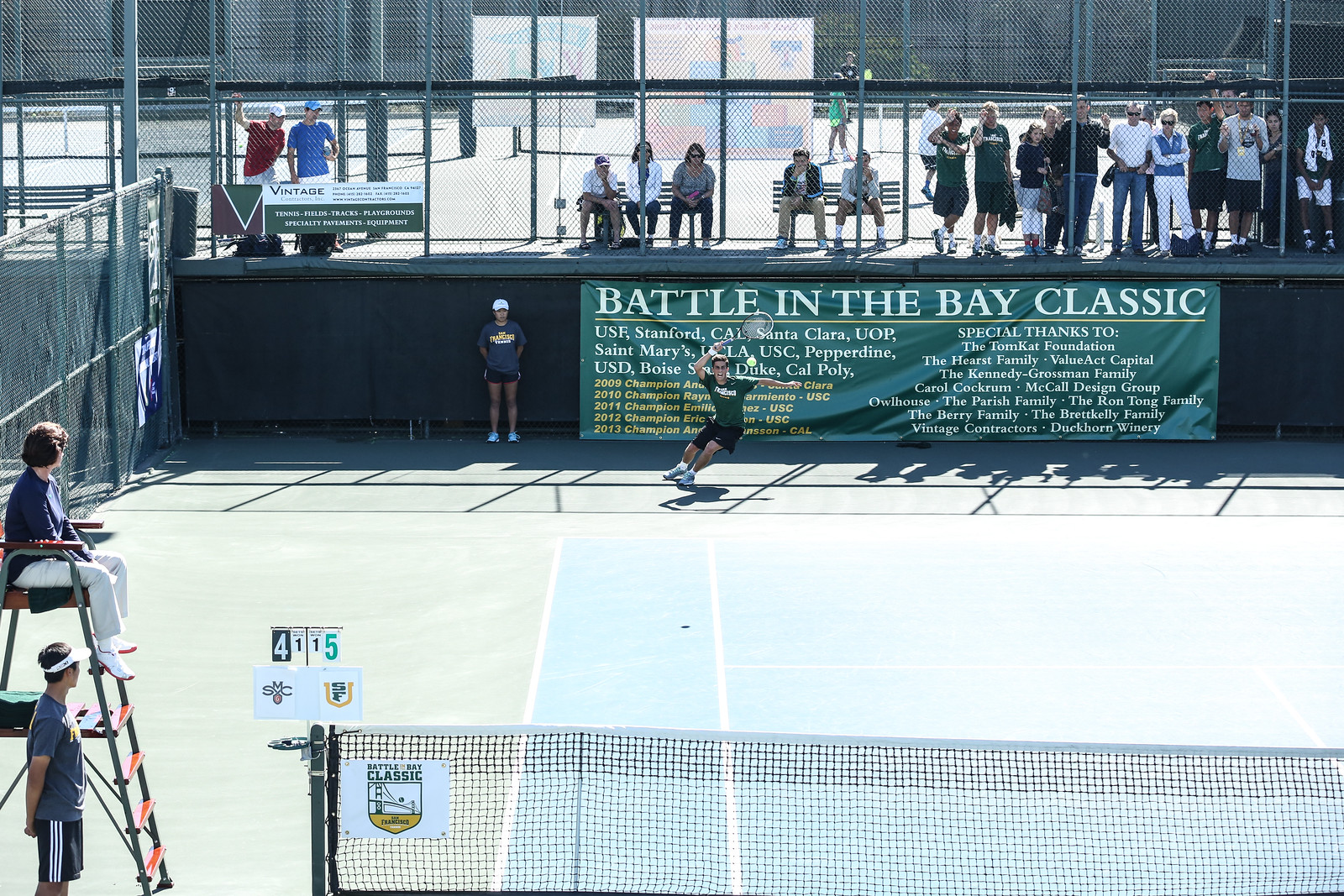This image captures an intense moment during a tennis match at the outdoor "Battle in the Bay Classic." In the foreground, a man in a green shirt and black shorts is poised to return an incoming ball, his tennis racket raised high above his head. The net prominently defines the front of the scene. To the left, a female umpire is seated in her high chair, attentively observing the game, while a ball boy stands ready beside her, prepared to retrieve the ball. Behind the player, a linesperson is positioned against a dark background. The green court, adorned with crisp white lines, contrasts with the vibrant green banner in the background that reads "Battle in the Bay Classic," listing prestigious universities such as USF, Stanford, Santa Clara, UOP, St. Mary's, USC, Pepperdine, USD, Boise, and Duke. The banner also acknowledges past champions from 2009 to 2013, along with various sponsors under "special thanks." Elevated in the background, spectators either stand or sit on benches, intently watching the match unfold. The current score indicates a closely contested game, tied at one set apiece, with the match standing at five to four.